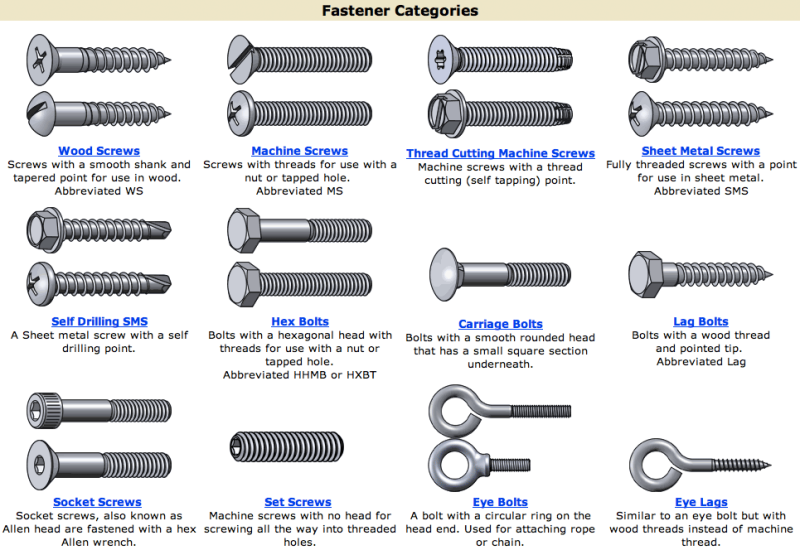The landscape-oriented image is an informational page titled "Fastener Categories," prominently displayed in a narrow beige band with black text at the top. The content below this heading is a detailed list of various fasteners, mainly screws and bolts, arranged in three rows. Each fastener type is paired with a CAD-generated illustration above its name, which is in bright blue text resembling clickable URLs. Below each name, in smaller black text, is a brief description of the fastener. The first row features wood screws, machine screws, and thread-cutting machine screws. The second row showcases sheet metal screws, self-drilling SMS screws, and hex bolts. The third row includes carriage bolts, lag bolts, socket screws, set screws, and a pair of eye bolts. The illustrations are computer-generated models that clearly depict the different head shapes, such as Allen head, flat head, hexagon, and rounded, and some fasteners have hooks or eyes. The detailed arrangement and black-and-white illustration style with accompanying text provide a comprehensive overview of 12 types of fasteners, each meticulously categorized and described.